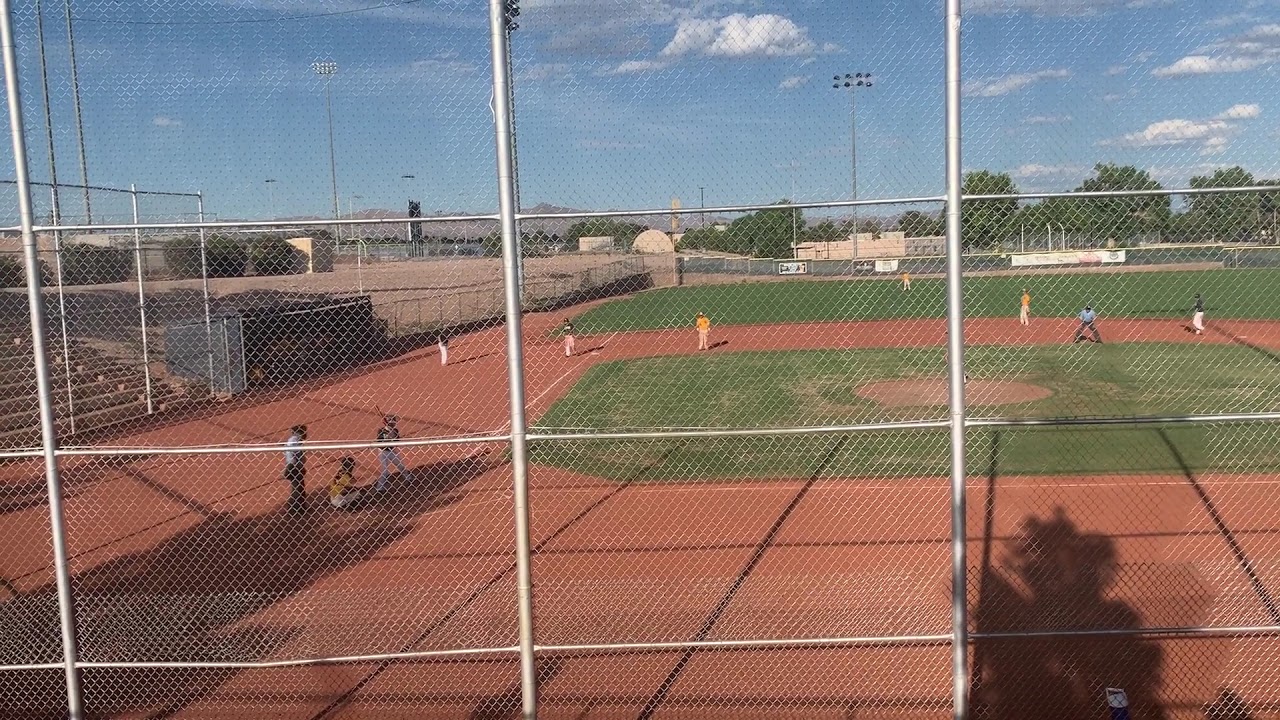This photograph captures a vibrant scene at a baseball diamond on what appears to be a beautiful spring or summer day. The image is taken from behind a silver chain-link fence, designed to keep baseballs from flying into the audience. The field itself is a mix of red dirt and green grass, with distinct areas of each visible both infield and outfield. At the center of the action, a young batter is poised to swing, with a baseball bat raised behind his head. Behind him, the catcher is in a crouched position, and standing just behind the catcher is the umpire. The outfield also features a few players ready for action. In the distance, stadium lights tower over the field, and beyond, there are trees and some buildings. The sky above is a clear blue with a few scattered white clouds, emphasizing the bright and pleasant weather. There are no visible spectators in the stands, suggesting this could be a practice session. Shadows cast by the players and the fences highlight the time of day, reinforcing the lively and warm atmosphere of the scene.